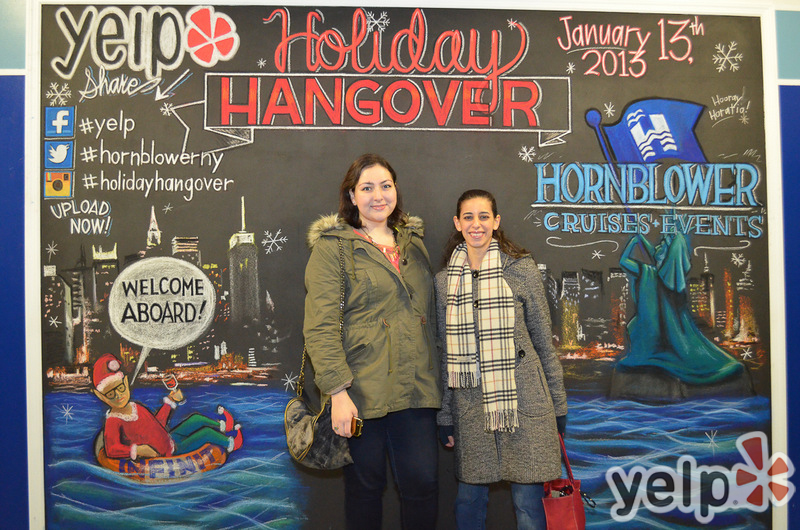The picture features two women standing in front of an intricately decorated mural that serves as an advertisement for a Yelp event. The mural, which resembles a colorful chalk drawing, prominently announces "Holiday Hangover, January 13th, 2013" and "Hornblower Cruises and Events" at the top. The design includes a whimsical illustration of the Statue of Liberty blowing a horn labeled "Hooray Horatio," as well as a snow-covered cityscape filled with skyscrapers and a river scene. An elf dressed like Santa is depicted floating in a tube labeled "Infinity," and he holds a glass of wine while saying, "Welcome Aboard." Social media icons and hashtags such as #Yelp, #HornblowerNewYork, and #HolidayHangover invite viewers to share and upload pictures. The Yelp logo appears in the upper left and lower right corners of the mural. In front of this vibrant backdrop, the two women are smiling for the camera. The woman on the left wears a heavy green jacket with a fur collar, an orange blouse, blue pants, and a handbag over her right shoulder. The woman on the right is dressed in a long gray coat, blue jeans, and a white and blue striped scarf, with a purse in her left hand. Both are bundled up warmly, suggesting it is a cold day.